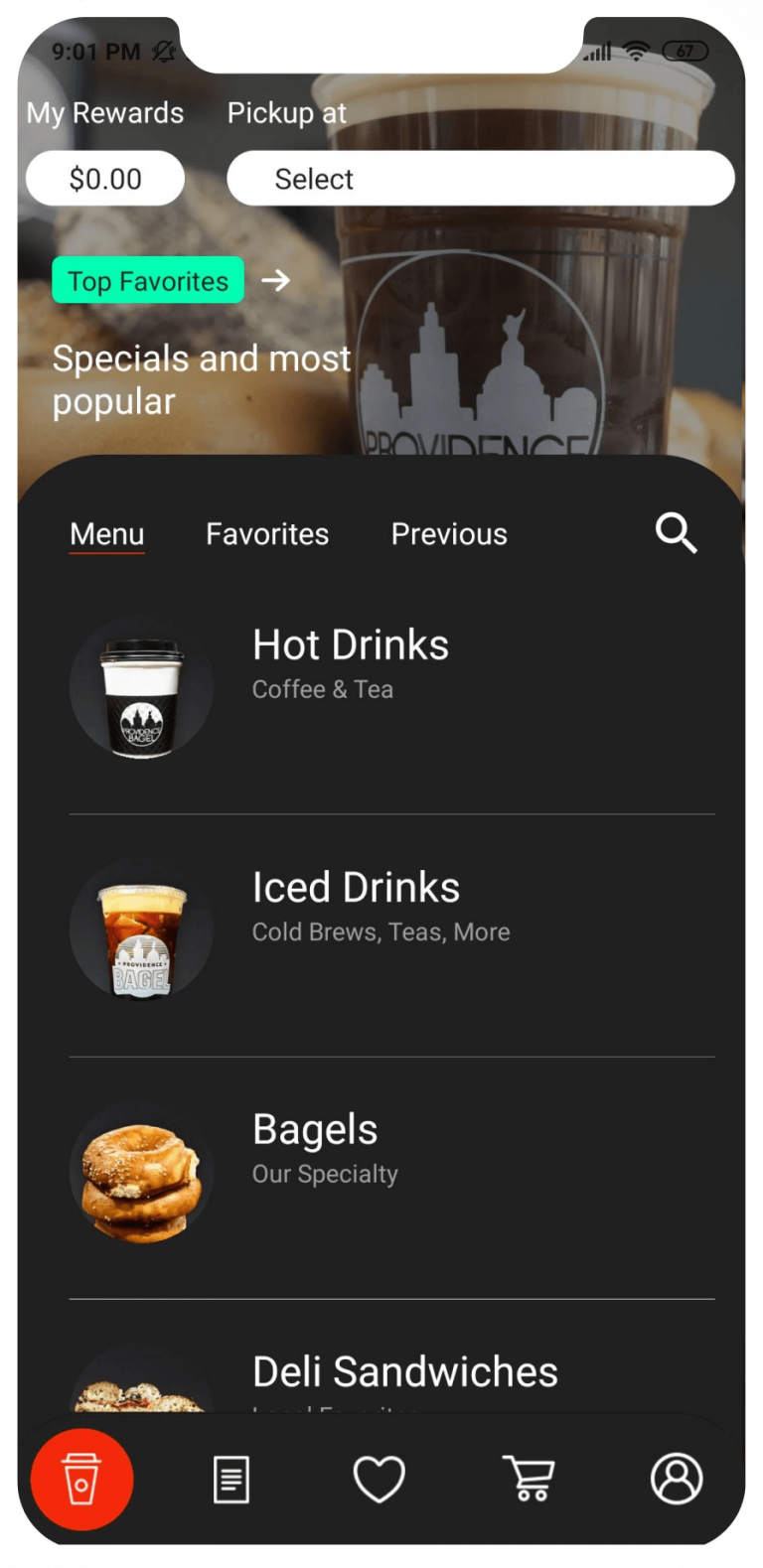This screenshot captures the user interface of an app designed for managing rewards and placing pickup orders. At the top left corner, the interface displays "My Rewards" with the current balance set to $0.00. Adjacent to this, there's a section labeled "Pickup" with an unselected drop-down bar indicated by the word "Select."

Directly below, a section with a green rectangular background and black text reads "Top Favorites." Followed by this are two additional sections labeled "Specials" and "Most Popular." Further down, the interface features three tabs titled "Menu," "Favorites," and "Previous," with the "Menu" tab currently active.

Within the "Menu" tab, the first category visible is "Hot Drinks," encompassing "Coffee and Tea," "Ice Drinks," and "Cold Brew." Next, there's a section for "Bagels" labeled "Our Specialty." The final visible category is "Deli Sandwiches," but the text beneath it is cut off, preventing further details from being seen.

At the bottom navigation bar of the app, icons are present: a heart symbol in the middle, a cart symbol on the left, and a stick figure icon on the far right, which presumably takes the user to their profile when clicked.